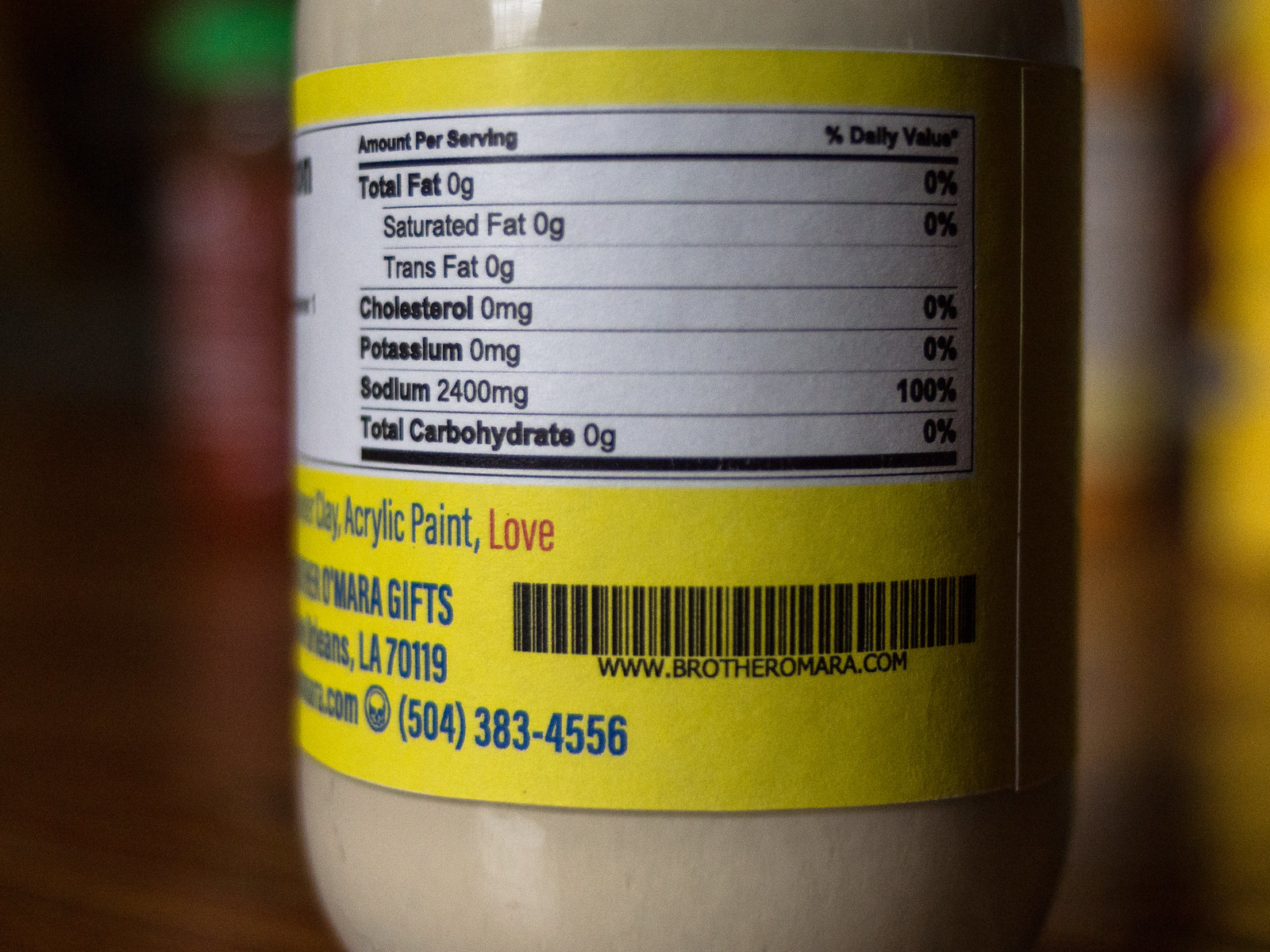This image features a bottle of acrylic paint prominently positioned in the foreground, partially cropped at the bottom to obscure the base. The bottle appears to rest on a flat surface such as a table or desk. In the background, several out-of-focus bottles are visible, providing context to the environment.

The acrylic paint bottle in question has a light hue, somewhere between white and beige. The label is distinctive, bordered in yellow, and features detailed nutritional information traditionally found on food packaging. It lists "Amount per serving: Total Fat 0g, Saturated Fat 0g, Trans Fat 0g, Cholesterol 0mg, Potassium 0mg, Sodium 2400mg, Total Carbohydrate 0g."

Ingredients are also specified: "Acrylic Paint," noted in blue letters, and the word "Love," highlighted in red letters. At the bottom of the label, contact information is provided: "Mar Gifts LA 70119," a barcode with the website "www.brothermara.com," and a phone number in blue text: "504-383-4556."